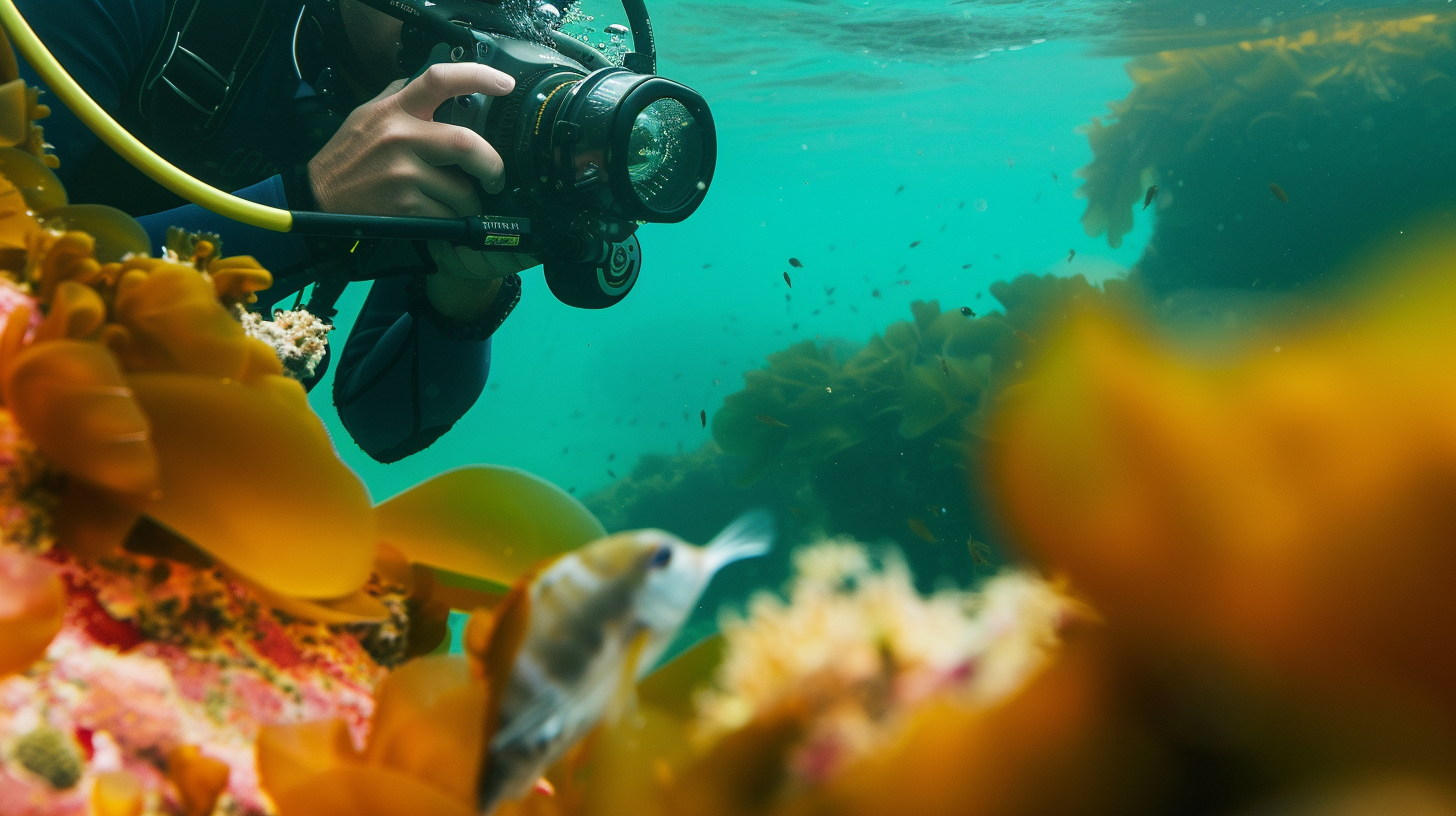In this vibrant underwater photograph, a scuba diver is captured in the midst of taking pictures of the rich sea life around them. The diver, clad in a blue-sleeved shirt and a black dive suit, is seen in the upper left portion of the image, holding a black and yellow camera up to their face. Notably, they are using a clear glass mask and a black and yellow breathing hose. 

The foreground of the image provides an intricate view of the seafloor adorned with various types of coral, showcasing vivid hues of orange, yellow, pink, and white. Amidst the colorful scene, a small fish with yellow stripes and a long nose is prominently visible, adding a sense of scale and detail to the photograph. There's also a blurred view of some seaweed and sea kelp in the background, indicating the diverse marine ecosystem. 

Overall, the image captures the interplay of vibrant marine life set against the serene blue-green expanse of the ocean, framed by the focused presence of the scuba diver engrossed in their underwater photography.